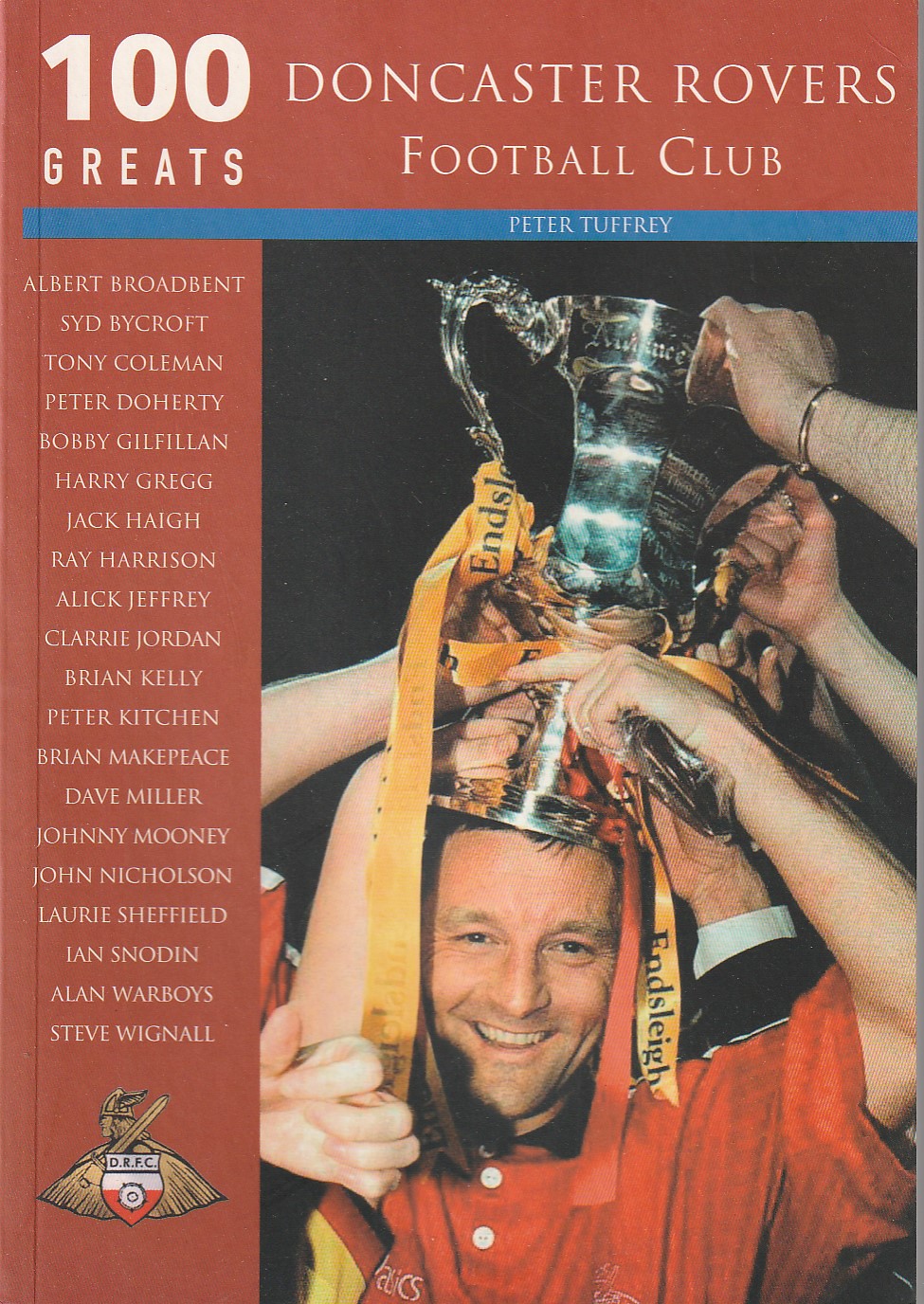The cover of a red magazine features a striking image of a man in a red shirt holding a silver trophy with a yellow ribbon above his head, surrounded by multiple hands reaching out to touch the trophy. This image is positioned on the right side of the cover, extending from the bottom right well above the center. The man is smiling, encapsulating a moment of shared triumph.

At the top, bold white text reads, "100 Greats, Doncaster Rovers Football Club." Along the left-hand side is a comprehensive list of notable names associated with the club, including Albert Broadbent, Sid Bycroft, Tony Coleman, Peter Doherty, Bobby Gilfoyan, Harry Gregg, Jack High, Ray Harrison, Alec Jeffery, Claire Jordan, Brian Kelly, Peter Kitchen, Brian Makepeace, Dave Miller, Johnny Mooney, John Nicholson, Laurie Sheffield, Ian Snowden, Alan Warboys, and Steve Wignall. 

Additionally, there is a small blue bar with the name "Peter Tuffrey" in it. Below the list of names, the Doncaster Rovers Football Club logo is depicted, showcasing a shield featuring a knight equipped with a helmet, cape, and sword.